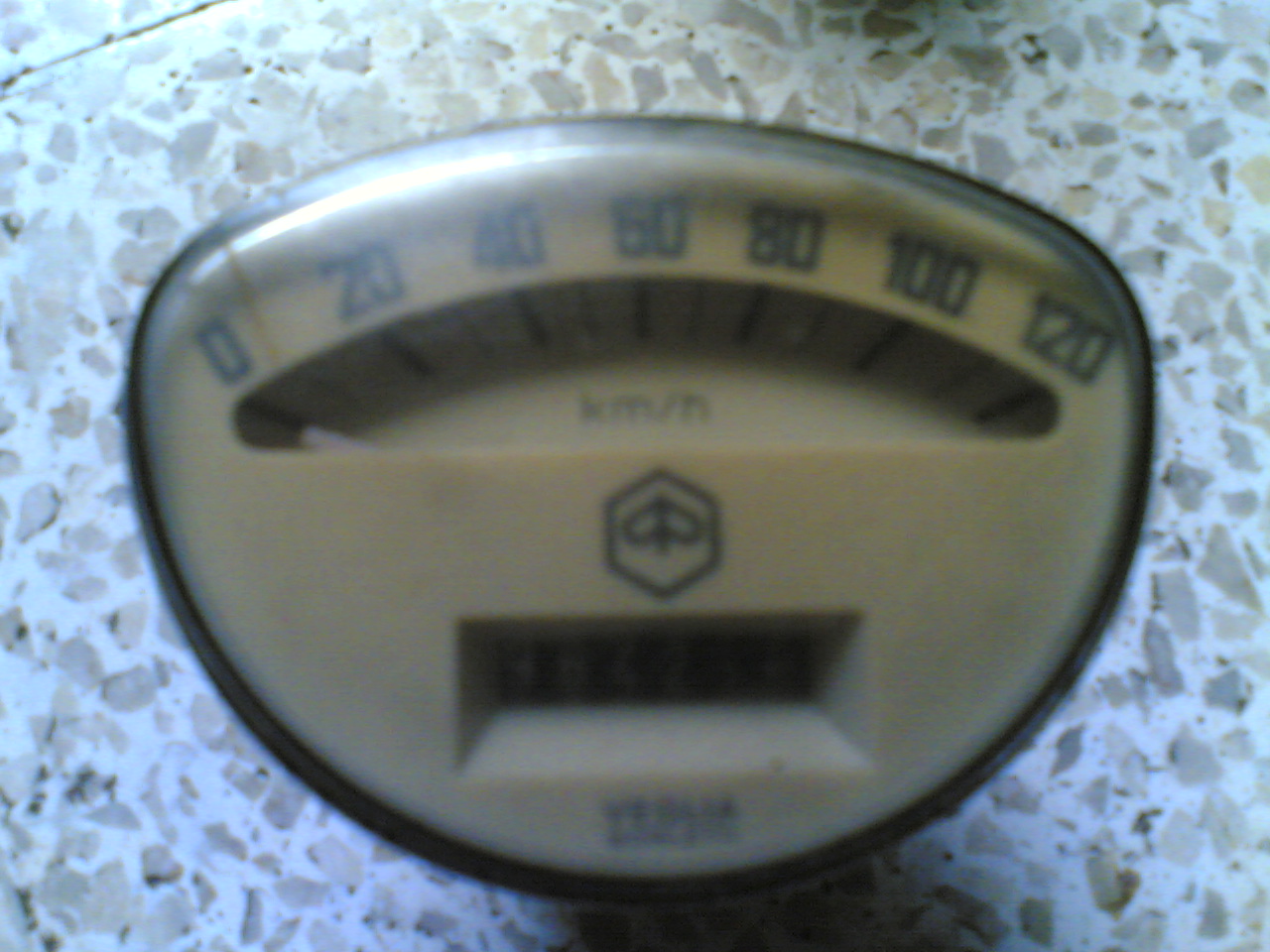A close-up image captures a device sitting prominently on a white counter table speckled with brown and beige. The device, bordered in black, features a light brown or beige background and is almost oval-shaped but squared at the top. It dominates the picture frame. At the top of the device, black numbers display increments of 0, 20, 40, 60, 80, 100, and 120. Beneath the numbers, an opening showcases several black lines, with a red line positioned slightly past the zero mark. The central section of the device features the inscription "KM-N," with a small hand resting on the first of 7 or 8 lines. There is also an octagonal emblem containing a smaller black emblem below this section. Towards the bottom, another open area shows some text, though it’s illegible. The entire device appears to be encased in a dome made of plastic or glass.